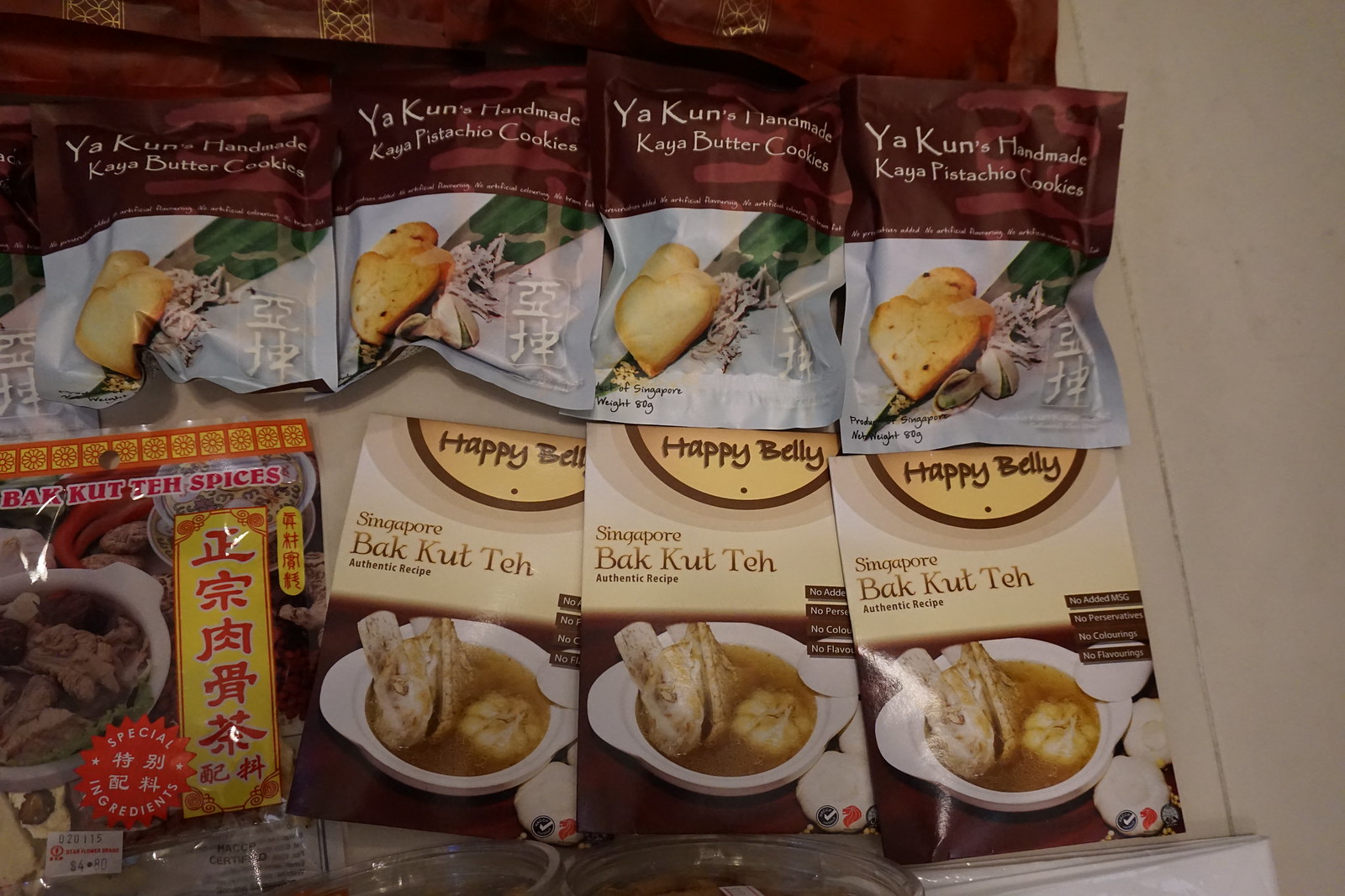The photo depicts a detailed display of various Singaporean or Chinese food items and authentic spices, likely staged in a Southeast Asian supermarket. Positioned prominently at the top is what appears to be dried vegetable roots, possibly potatoes, accompanied by pistachios. Below this, there are rows of spices labeled as special ingredients for soups, each emphasizing their authenticity with claims of "no added MSG, no preservatives, no colors, no flavoring." 

On the bottom left, there's a bag labeled "Bak Kut Teh" spices, associated with the brand "Happy Belly." This brand also offers a cookbook titled "Singapore Bak Kut Teh," showcasing traditional recipes. Beside these spices, another cookbook and bags of spice mix highlight the iconic Singaporean stew. To the right, upping the visual appeal, are packages of Yakun's handmade Kaya pistachio and butter cookies, distinctive with their oblong shape and displayed in vibrant yellow and red packaging.

The setup, neatly arranged against a white wall, underscores the diversity of the regional cuisine with its rich assortment of flavors and traditional staples, encapsulating a glimpse into authentic Singaporean culinary delights.